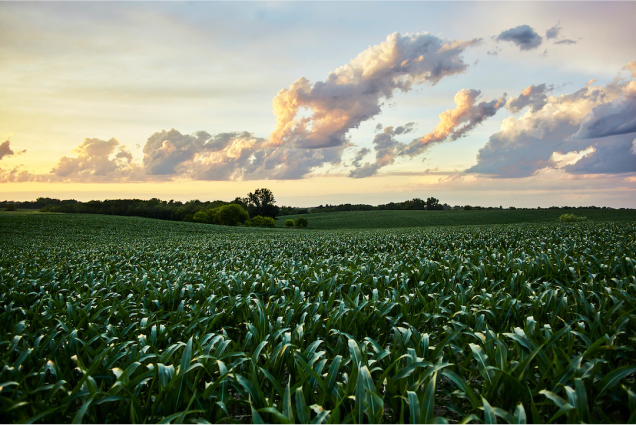Looking out over a vast field of vibrant, lush green corn, the endless rows of stalks create a mesmerizing patchwork that stretches as far as the eye can see. The scene is captured from a low-angle perspective, emphasizing the corn's height and dense arrangement, with some leaves curving down at the edges and others showing intricate veins of white and yellow. The sky above is a remarkable blend of pale blue and pink hues, scattered with wispy and puffy clouds that add texture and depth. The horizon reveals a contrasting landscape of a distant ridge lined with trees and light green shrubbery, hinting at the peaceful expanse beyond the cornfield. The subtle glow from the sun, possibly setting or just set, casts a serene light over the scene, creating a delicate interplay of shadows and highlights. In the far background, water glistens softly, adding to the tranquil ambiance of this expansive, pastoral vista.